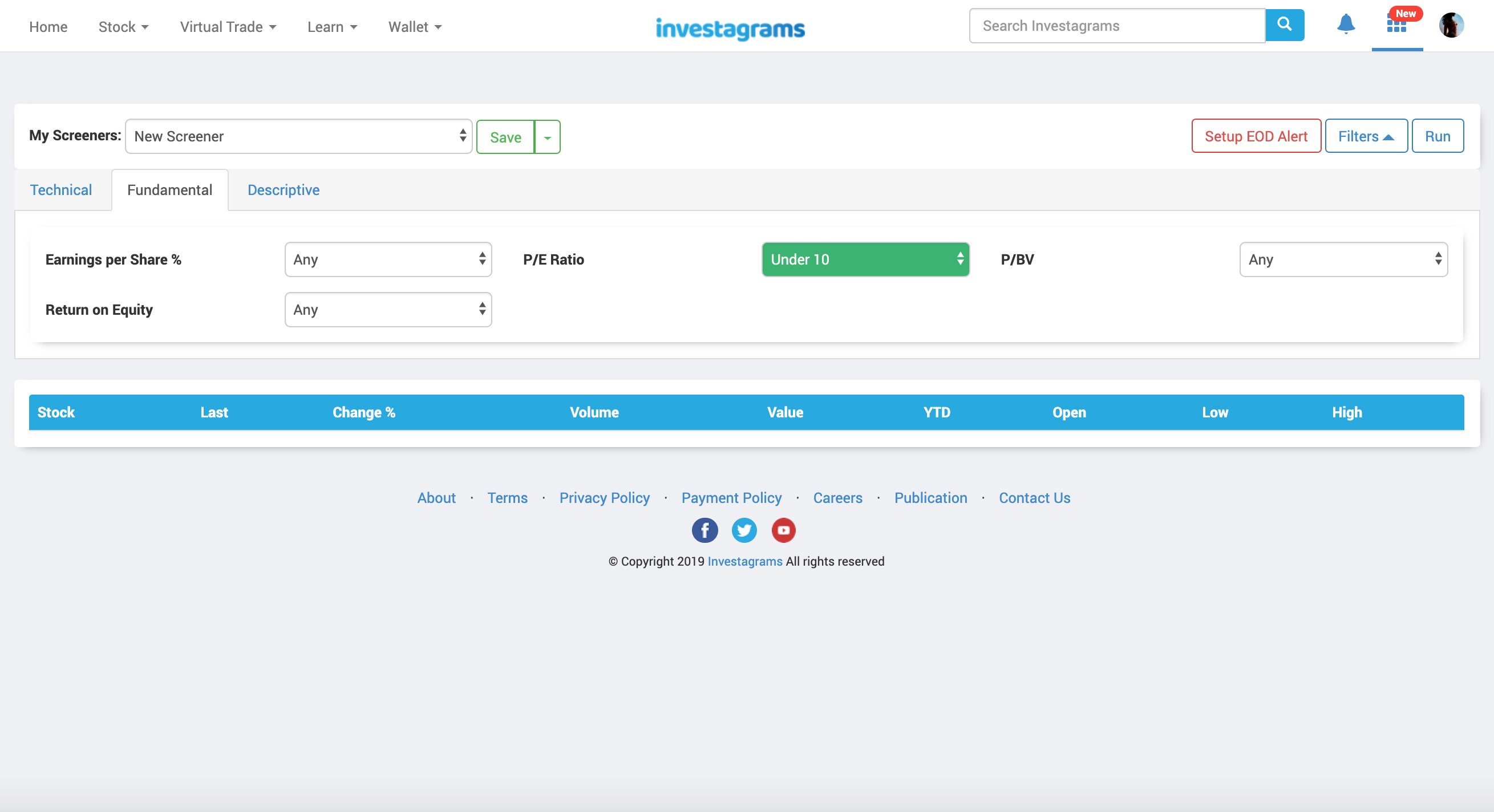The image depicts the homepage of the Investagrams website, showcasing a detailed layout of various features and functionalities. At the top of the page, the Investagrams logo is prominently displayed in blue. In the top left corner, several navigation tabs and drop-down options are visible, including 'Home,' 'Stock,' 'Virtual Trade,' 'Land,' and 'Wallet.' On the top right corner, there's a search bar labeled "Search Investagram," with a blue search icon, a blue notification icon, a 'Create' icon marked with a red "New" tag, and a 'Profit Page' icon.

In the center-left section of the page, the label "My Screeners" appears with a new screener option and a green 'Save' button. To the right, there is the 'Setup EOT' section featuring 'Filters' and 'Run,' both highlighted in blue. The left-center of the screen contains tabs labeled 'Technical,' 'Fundamental,' and 'Descriptive,' with 'Fundamental' highlighted in black while 'Descriptive' and 'Technical' are in blue. Below that, data points such as 'Earnings Per Share,' 'Return on Equity (ROE),' 'PE Ratio' and 'PBV Ratio' are listed, with interactive options to select various criteria.

At the bottom of the image, several stock metrics are shown, including 'Stock,' 'Last,' 'Change,' 'Volume,' 'Value,' 'YTD,' 'Open,' 'Low,' and 'High.' The footer of the page lists links to 'About,' 'Terms,' 'Privacy Policy,' 'Payment Policy,' 'Careers,' 'Publications,' 'Contact Us,' Facebook, Twitter, YouTube, and asserts the copyright of Investagrams dated 2019 with an "All rights reserved" note.